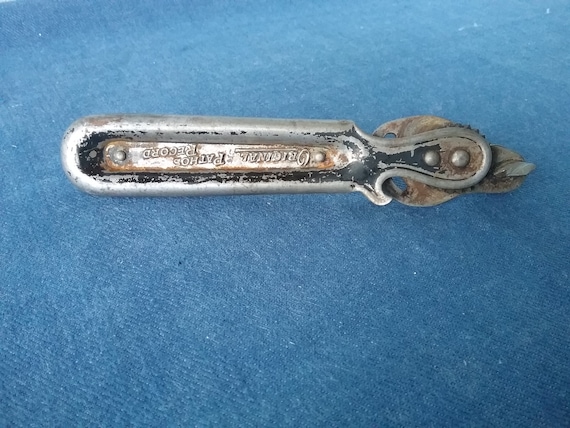This photograph features a prominently blue background that resembles a canvas or denim cloth. Laying on this surface is an aged, heavily rusted metal tool, most likely a wrench. The tool, originally a silver color, is encrusted with layers of rust varying from light brown to black. The right-hand edge of the tool curves around in a hook-like shape, almost resembling a bottle opener, and includes two small rivets. There is text engraved on the handle, though it is partially illegible due to the rust and dirt, with possible remnants reading "original patho record." Despite its blunted yet sharp appearance, the tool's specifics are obscured by the extensive wear and corrosion.